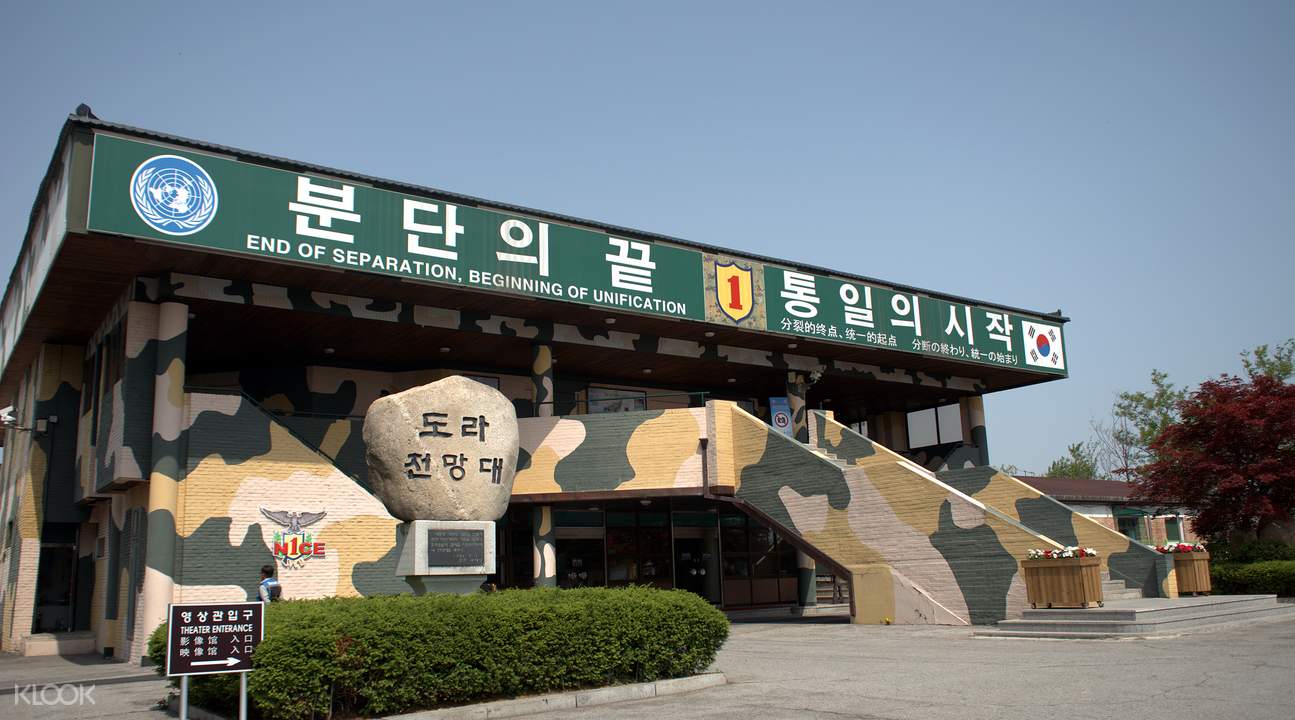This picture, taken outside, captures the front view of a building adorned in camouflage colors, featuring shades of white, tan, and green. The building stands on a gray cement foundation and is approached by a concrete stairway that leads up to the front door, spanning two stories. The camouflage design of the building extends to the stairway, blending in with shades of light brown, beige, and dark green. In front of the building, there is a green banner with white letters in both Asian (likely Chinese) and English, stating, "End of Separation, Beginning of Unification." 

On the left side of the green banner, there is a blue circle symbol resembling the United Nations logo, and to the right of the sign, there are additional Asian characters and a flag featuring a red and blue center. Centrally positioned on the building's facade is a golden yellow shield with a red number one. Below the banner, a long green bush extends horizontally. 

To the left, there's a small black and white sign with unreadable text, and a large rock with Asian writing serves as a monument. The right side of the facade displays potted plants in brown boxes containing red and white flowers and a stairway leading up. A clear, blue sky and several trees, including one with purple leaves, frame the building, contributing to the tranquil ambiance.